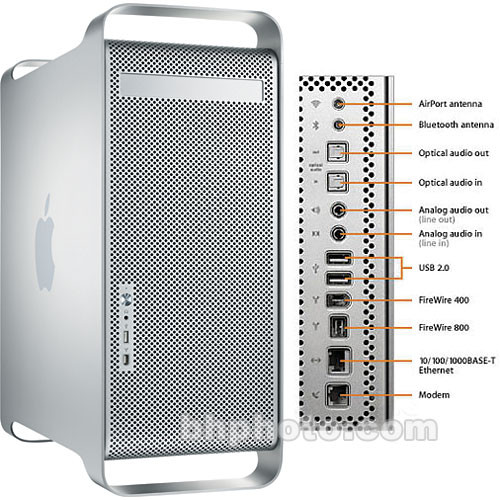Here is a detailed caption formed by merging and refining the three provided captions:

The image provides a detailed view of a silver Apple desktop computer against a white background, displayed in a square format with some digital enhancement. The left section of the image showcases the front of the computer, highlighting the power button and multiple USB ports. Prominently, the computer features the iconic grey Apple logo on its side - an apple with a leaf and a bite taken out of it.

The right section of the image illustrates the back of the computer, demonstrating various ports and inputs, each meticulously labeled. These include: an AirPort antenna, a Bluetooth antenna, optical audio out, optical audio in, analog audio out, analog audio in, USB 2.0, FireWire 400, FireWire 800, and a modem. The labels are written in neat black text adjacent to each corresponding port. Additionally, a faint watermark, reading "B-H-P-H-O-T-O-T .com," is visible across the bottom of the image.